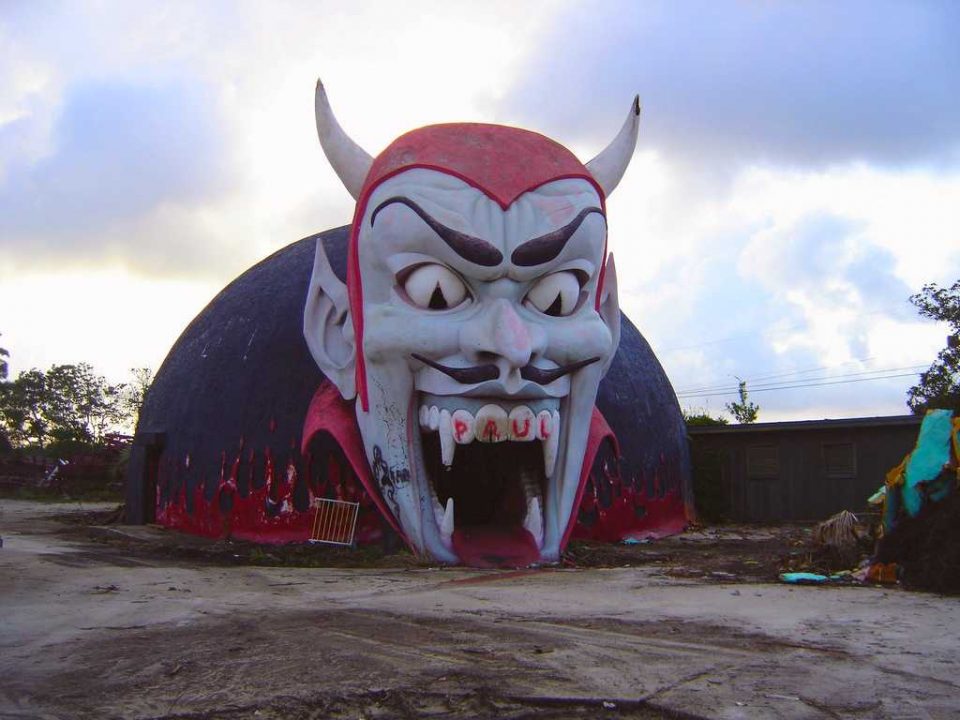This intriguing outdoor photograph, taken during the day under a mostly overcast sky, captures an eerie scene set against a nearly treeless backdrop, punctuated by a few minimal trees on either side. The foreground features an abandoned lot where the main focus is an inflatable dome structure. The dome is predominantly black with red flames along the bottom, enhancing its ominous appearance. The centerpiece of the structure is a menacing face that appears to be a hybrid between a devil and Dracula, complete with exaggerated fangs. Red letters spelling "Paul" are inscribed on the teeth, adding to the unsettling vibe. The mouth of this sinister figure is wide open, with a long tongue extending outward, inviting visitors to walk inside, reminiscent of an attraction one might find at a miniature golf course.